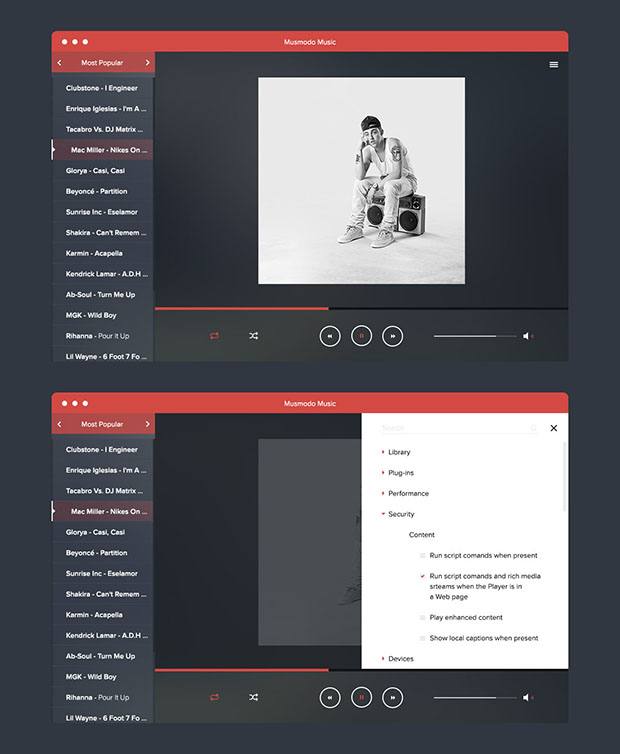This is a detailed screenshot depicting the Masumoto Music website. The page features a grayscale theme with dynamic accents in white and red. Centrally positioned, a striking black-and-white photo showcases a young man exuding a pensive mood. He sits atop a boombox with his head resting on his hand, wearing a backward baseball cap, a white tank top, jeans, sneakers, and sporting visible tattoos.

On the left side of the page, the heading "Most Popular" appears in bold red text. Below this, in white font against a black background, is a list of artists and bands such as Clubstone Engineer, Enrique Iglesias, Tacabro vs DJ Matrix, Mac Miller, Nike's, Glory's, Beyoncé, Sunrise Inc., Shakira, Carmen, Kendrick Lamar, Ab-Soul, MGK, Rihanna, and Lil Wayne.

Reiterating its branding, "Masumoto Music" appears again within a distinctive red bar. This section also repeats the list of popular artists mentioned earlier.

On the right, a white box contains various menu options including 'Library, 'Plug-ins,' 'Performance,' 'Security,' and 'Content.' Under these main categories are additional settings related to running script commands and media enhancements when the player is active on a webpage. This area is equipped with standard playback control icons such as play, pause, fast forward, and restart, contributing to a comprehensive media experience for the user.